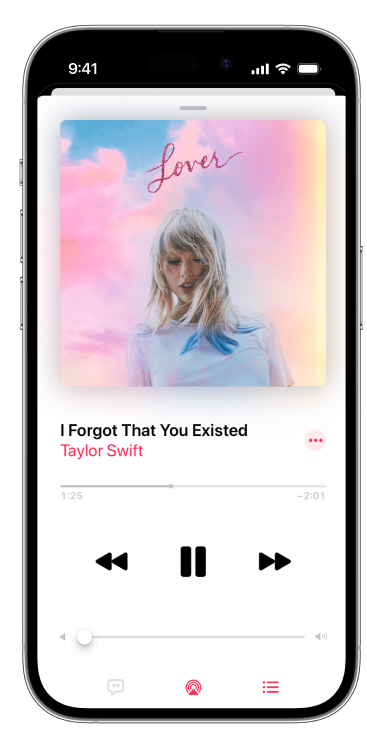The image depicts a prototype of a black smartphone displaying a music app interface. The top of the phone screen shows the current time as 9:41 in white lettering, along with indicators for cellular signal strength, Wi-Fi connectivity, and battery life.

The main focus of the screen is the music app, currently featuring an album cover of Taylor Swift's "Lover." The background of the album cover shines in shades of pink, light orange, and yellowish clouds. In the image, Taylor Swift gazes downward with part of her hair, tinted blue at the tips, falling slightly over her face. She is adorned in a white shirt, and above her head, the word "lover" is elegantly inscribed in pink.

Beneath the album cover, the song title "I Forgot That You Existed" is displayed in black lettering, with "Taylor Swift" written in red beneath it. The track's progress bar indicates the song is 1 minute and 25 seconds into play, with a time remaining of -2:01 seconds, implying the song’s conclusion.

Below the progress bar, centralized controls for the music player are evident. The play/pause button is represented by two dark, vertical black lines. To its left is the black rewind symbol, and to its right, the black forward symbol, both characterized by arrows pointing in opposite directions. Further down, a volume adjustment bar is visible, featuring a movable white circle for volume control.

At the bottom of the screen, there are additional icons: a small chat-like icon (details unclear), a red antenna-like symbol, and three horizontal red lines each paired with a trio of dots, presumably representing additional settings or controls.